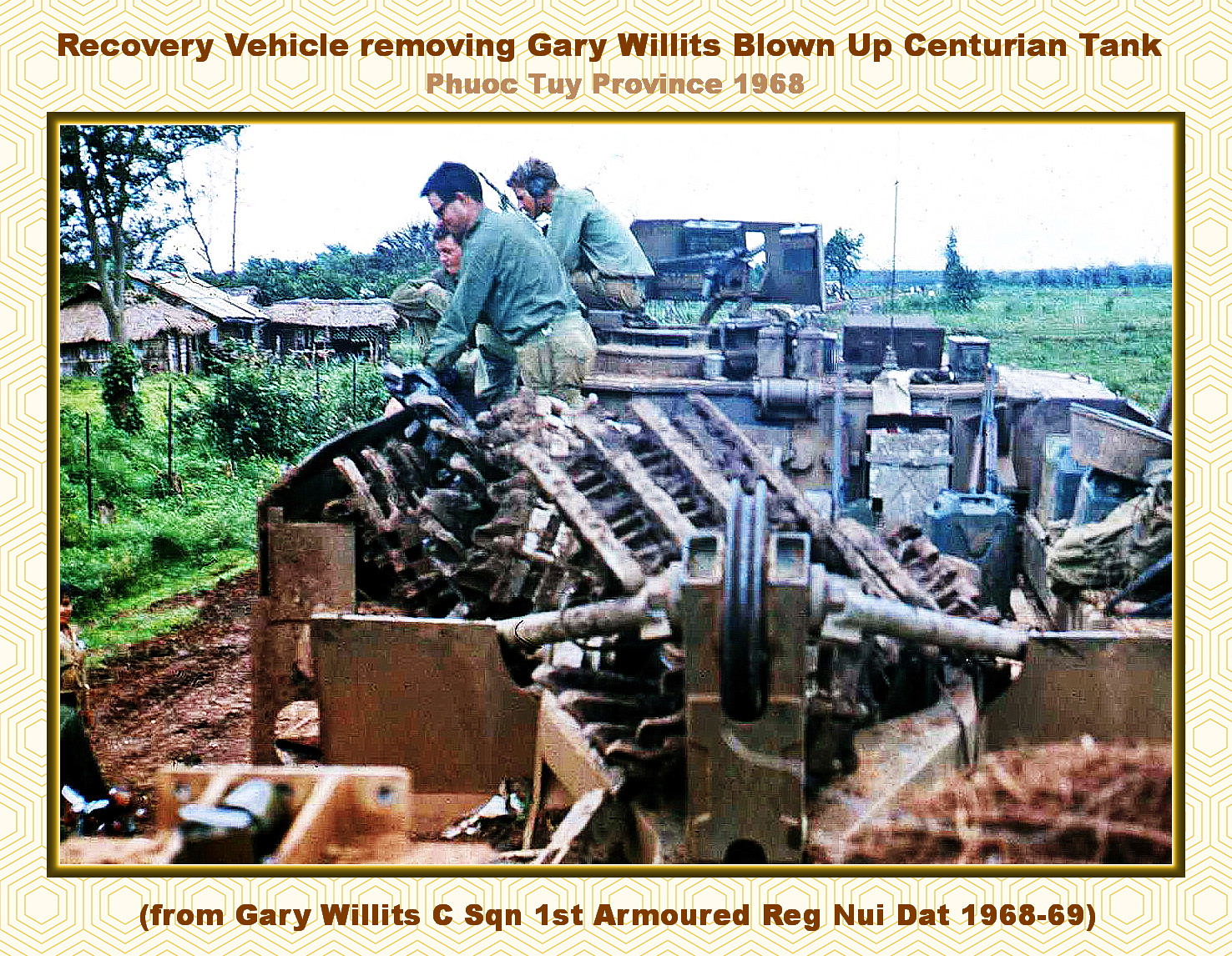This photograph, taken in Phuoc Tuy Province, Vietnam, in 1968, depicts the recovery of Gary Willett's destroyed Centurion tank by a recovery vehicle. The image captures three men prominently positioned on the tank's remains. Standing within the interior of the visibly damaged tank is a man in a green shirt and camouflage pants. On top of the tank sits another man in a similar uniform, while a third individual in a green jacket stands between them. Various military gear, including a pulley system, can be seen in the truck, alongside buckets, cans, and fragments of metal. The backdrop features a series of huts with gabled roofs, verdant grass, and trees under an overcast sky. The photograph is bordered by text; the top reads, "Recovery vehicle removing Gary Willett's blown-up Centurion tank, Phuoc Tuy Province, 1968," while the bottom states, "From Gary Willett's C-Squadron, First Armored Regiment, 1968-69."